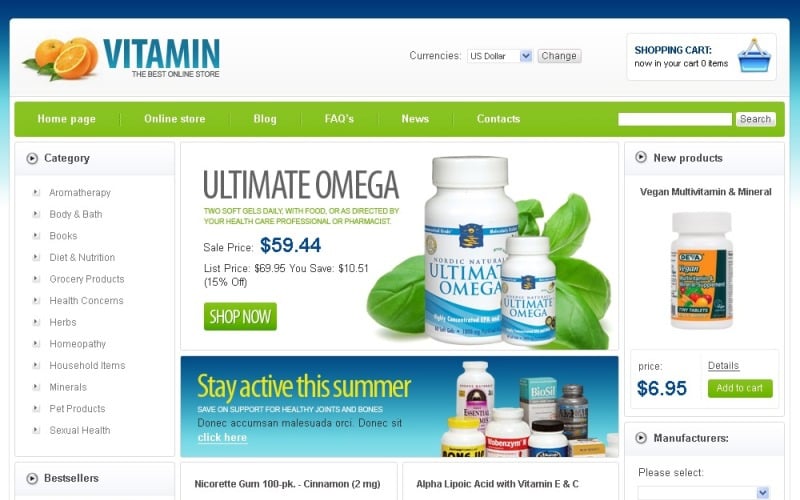The screenshot displays a well-organized online store interface. The top left-hand corner features an image of three oranges—two whole and one cut in half. Adjacent to this image are the words "Vitamin - The Best Online Store". 

On the right side, there is a prominent navigation bar containing a drop-down menu labeled "Currencies", currently set to USD. Next to it are a "Change" button and a shopping cart icon. Directly below, a vibrant green bar houses primary navigation links such as "Home Page", "Online Store", "Blog", "FAQs", "News", and "Contacts", with a search bar positioned beneath them.

To the left-hand side, beneath the green navigation bar, a vertical menu lists various categories including aromatherapy, body and bath, books, diet and nutrition, grocery products, health concerns, herbs, homeopathy, household items, minerals, pet products, and sexual health. Below this, another menu labeled "Bestsellers" is displayed.

The main section of the screenshot prominently features a couple of bottles of Ultimate Omega pills on sale, with a "Shop Now" button. Beneath this is an advertisement banner encouraging users to "Stay Active This Summer" with a clickable "Click Here" link and an assortment of various pills in different sized bottles and boxes depicted.

On the right-hand side, a product listing for a bottle of vegan multivitamin minerals is shown, complete with a price, a "Details" link, and an "Add to Cart" button. Below this section, the site prompts users to select from various manufacturers.